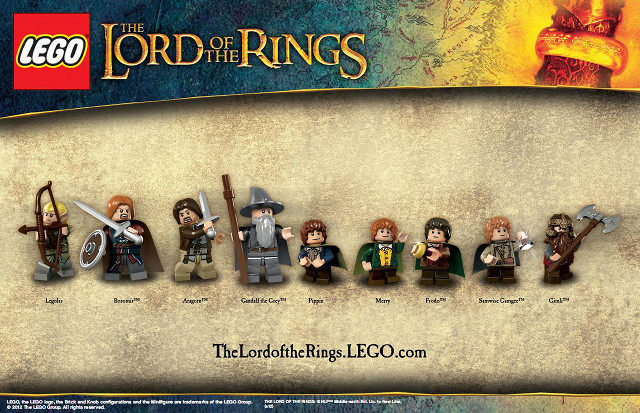This is a detailed photograph of a Lego box featuring characters from the Lord of the Rings franchise. The box prominently displays the Lego logo in white text on a red background in the upper left-hand corner. Adjacent to the logo is the iconic Lord of the Rings title, rendered in gold lettering, with a bright golden ring prominently featured on top of the scene.

The box showcases nine distinct Lego characters from the Lord of the Rings series, all lined up in a row against a cream-colored background with shadings of black and darker brown, which helps to accentuate the figures. Among the characters are a few holding different medieval weapons: one with a bow and arrow, another with a sword and shield, a wizard with a hat and staff, and four smaller figures each with different shades of brown hair. Another character holds a medieval weapon.

Despite the small print, the text "the lord of the rings.lego.com" is visible beneath the characters, with each character’s name printed underneath their respective figure. The overall scene is designed with dark colors typical of the Lord of the Rings aesthetic, making the box a very detailed and charming collectible set.